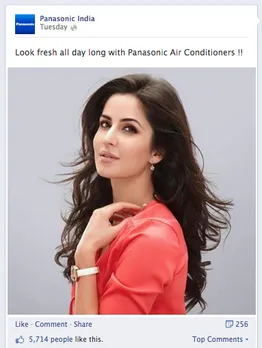This is a screenshot of a Facebook post from Panasonic India. The profile picture on the left features a blue square with white text. The post is timestamped "Tuesday" with a globe icon indicating its public visibility. A dividing line separates the timestamp from the main content. The text of the post reads, "Look fresh all day with Panasonic air conditioners."

Below the text, there is a photograph of a woman with long brown hair that reaches the middle of her back. She is positioned to the right side of the image, touching her neck with one arm. She is wearing a pink or salmon-colored shirt. 

The post includes interactive options such as "like," "comment," and "share" buttons beneath the photo. On the right side, it shows "256 comments" and the statement "5,714 people like this." The background of the post is gray at the bottom and white at the top.